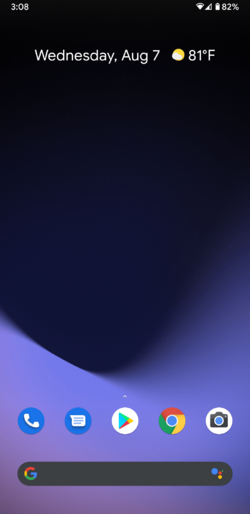This screenshot captures a smartphone display with intricate details. In the top-left corner, "3:08" is displayed in a small white font, indicating the current time. Proceeding right, a Wi-Fi symbol shows about 80% signal strength, followed by a signal strength indicator displaying two out of four bars. Further right, a nearly full battery icon is accompanied by "82%" in white lettering.

The background transitions elegantly from almost black at the top to dark purple, culminating in a light purple abstract design with a curved, ombre effect at the bottom. At the top of the screen, text displays "Wednesday, AUG 7," with "AUG" abbreviated. Adjacent to this, a sun icon with a cloud denotes the weather, alongside "81°F."

At the bottom, five icons are arranged in a row. From left to right, there is a blue circle with a white phone icon, a blue circle with a white message icon, the classic Play Store icon in a circle, the Chrome browser icon in a circular frame, and a circular camera icon.

Below these icons is an elongated oval search bar with a dark gray background. On the left side of the search bar is the multicolored Google "G," transitioning from red at the top to yellow, green, and blue. To the right are additional colorful dots: a large blue circle, and smaller red, yellow, and green circles.